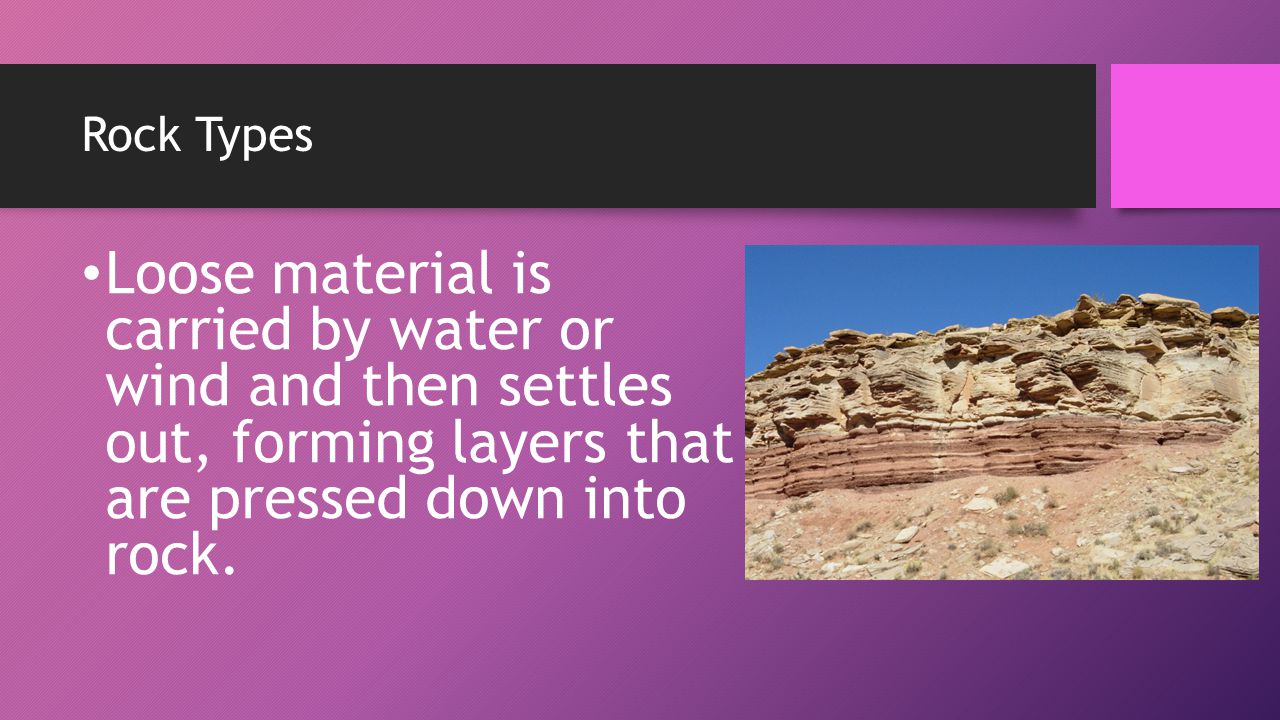The PowerPoint slide, with a background that transitions from light pink on the left to a darker, purplish hue on the bottom right, features a thick black banner at the top. This banner, adorned with white text reading "Rock Types" and a small bright purple square on the right-hand side, introduces the slide. Below the banner on the left side, a bullet point describes how loose material is carried by water or wind, settles out, and forms layers that are eventually pressed into rock. To the right of this text, an image of a cliff wall and a hillside showcases a stratified rock face, indicative of weathering, under a bright blue sky, with visible debris and scattered desert plants below. The contrast between the text's description and the visual representation provides a clear understanding of rock layer formation and weathering processes.